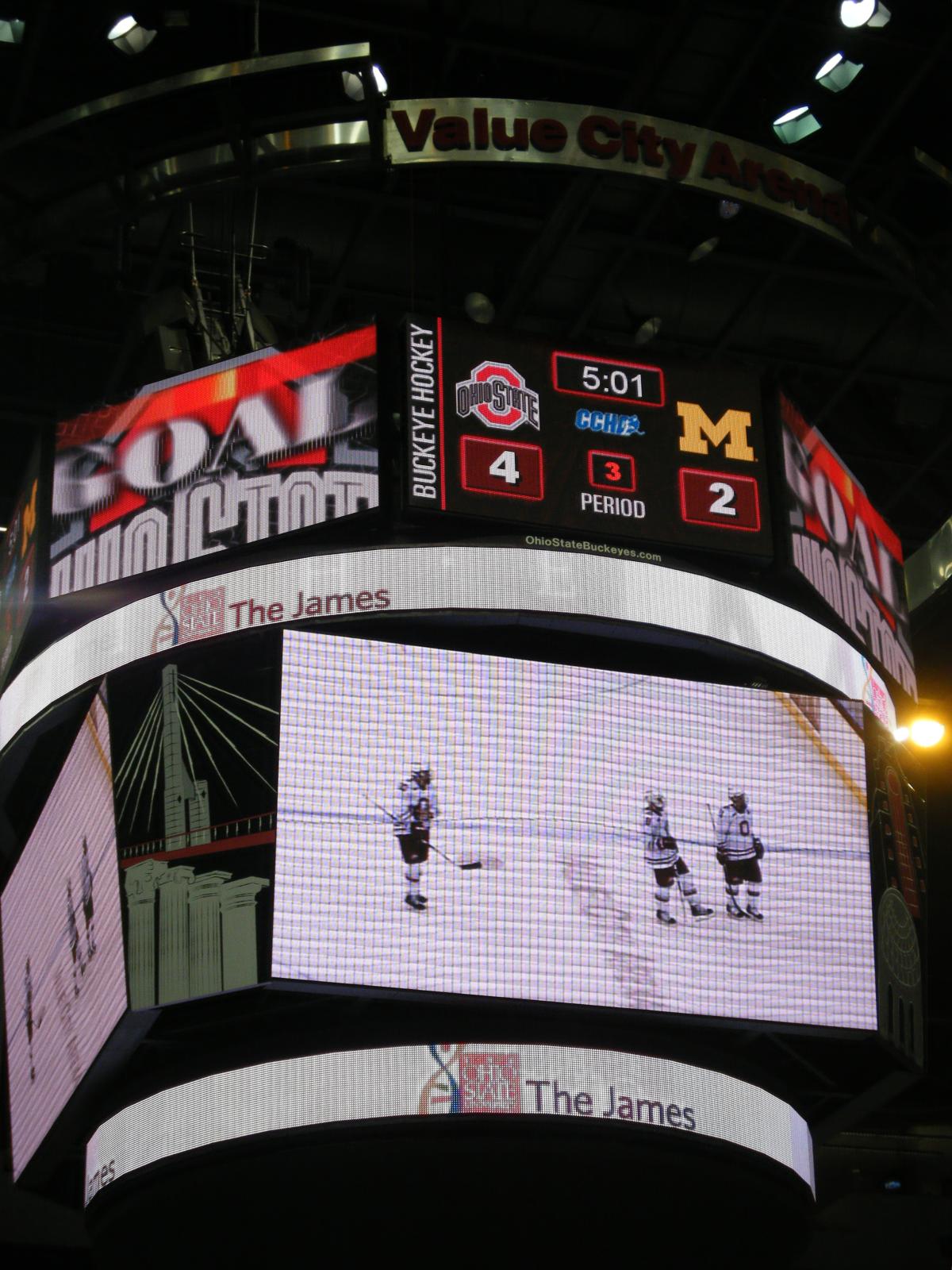The color photograph, taken in portrait orientation within a darkened Value City Arena, captures a detailed scene of a hockey game. Dominating the image is a scoreboard hanging over the middle of the ice rink, showcasing the words "Buckeye Hockey" and the score "Ohio State 4, Michigan 2," with 5:01 remaining in the third period. Above the scoreboard, a silver arc displays "Value City Arena," and beneath it, green and white signage reads "The James." The center of the scoreboard features an LCD screen displaying three hockey players on the ice, dressed in white jerseys and black shorts, each holding a hockey stick and appearing to look towards an unseen point. Additionally, the sides of the scoreboard feature the partially obscured word "goal," enhancing the game's dynamic atmosphere. The photographic representationalism style adds a layer of realism, immersing viewers into the live-action moment of the sporting event.